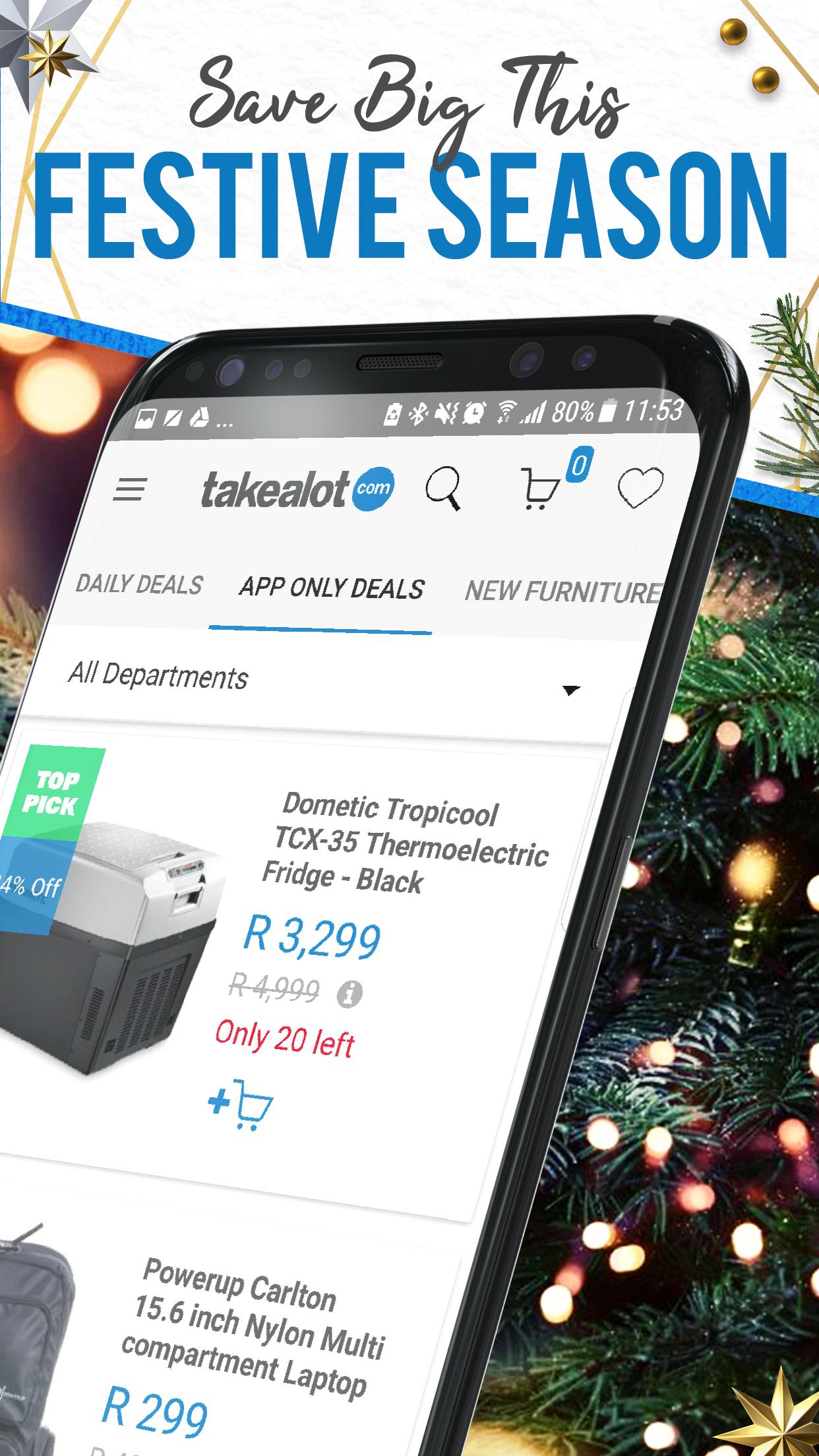This screenshot captures an advertisement on a cell phone, clearly designed to fit a cell phone's screen dimensions. The advertisement appears to promote holiday deals from Takealot, as indicated by the prominent display of the website's name on a picture of a cell phone within the ad. The backdrop of the ad features a festive Christmas tree adorned with glowing lights that extend back into the branches and hang below them, complemented by small golden stars sprinkled around the scene. The slogan "Save Big This Festive Season" is displayed at the top of the ad, with "Save Big This" in black font and "Festive Season" in an even larger, striking blue font. The front of the ad showcases a shopping interface on takealot.com, displaying a couple of highlighted products. The overall ambiance of the advertisement is festive, aiming to entice customers to take advantage of holiday savings.